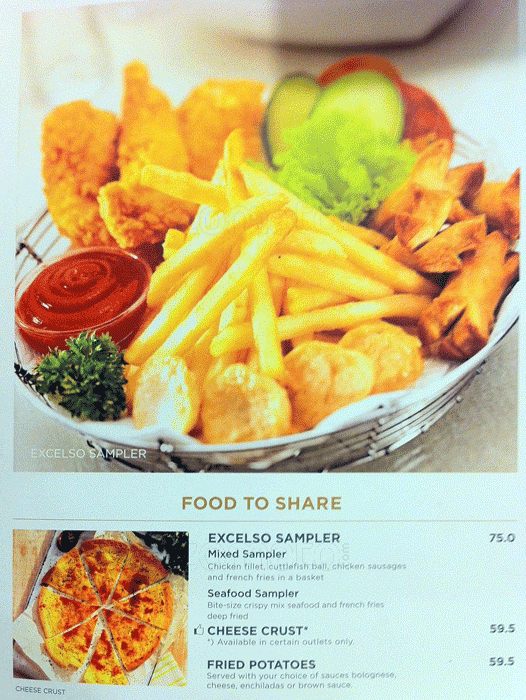The photo depicts a menu card against a light blue background. At the top half of the card, there is a large photograph showcasing a food basket filled with French fries, chicken fillets, chicken tenders, cuttlefish balls, and a cup of red sauce, garnished with fresh parsley. This basket, labeled "Excelso Sampler," features an assortment of fried items and is priced at $75. Below this image, the title "Food to Share" is prominently displayed.

To the left, there is a picture of a pizza sliced into eight pieces. On the right, the menu lists four items along with their prices: "Excelso Sampler - $75.00" which contains a mix of chicken fillet, cuttlefish balls, chicken sausages, and French fries; "Seafood Sampler" which includes bite-sized pieces of crispy mixed seafood and French fries, all deep-fried; "Cheese Crust - $59.50" available only at certain outlets; and "Fried Potatoes - $59.50" served with a choice of sauces including Bolognese, cheese, enchiladas, or brown sauce.